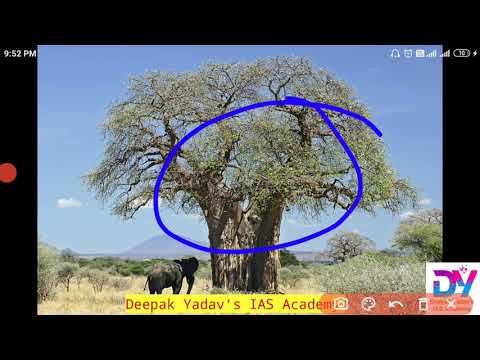The image is a screenshot displayed on a cell phone or tablet, showing a photograph of a sparse, massive tree with a wide trunk and wiry branches set against a clear blue sky. The tree, circled in a blue hand-drawn circle, provides shade for an elephant standing beneath it, suggesting a hot afternoon in an African safari-like setting, with scattered shrubs and bushes in the background. The screenshot frame includes a black border with a red dot on the edge. At the top of the screen, the time reads 9:52 PM in white, with battery and signal indicators on the right. Beneath the photo, a yellow strip with red text reads "Deepak Yadav's IAS Academy," accompanied by various editing icons such as a camera, painter’s palette, a back arrow, and an X on a faded red background.